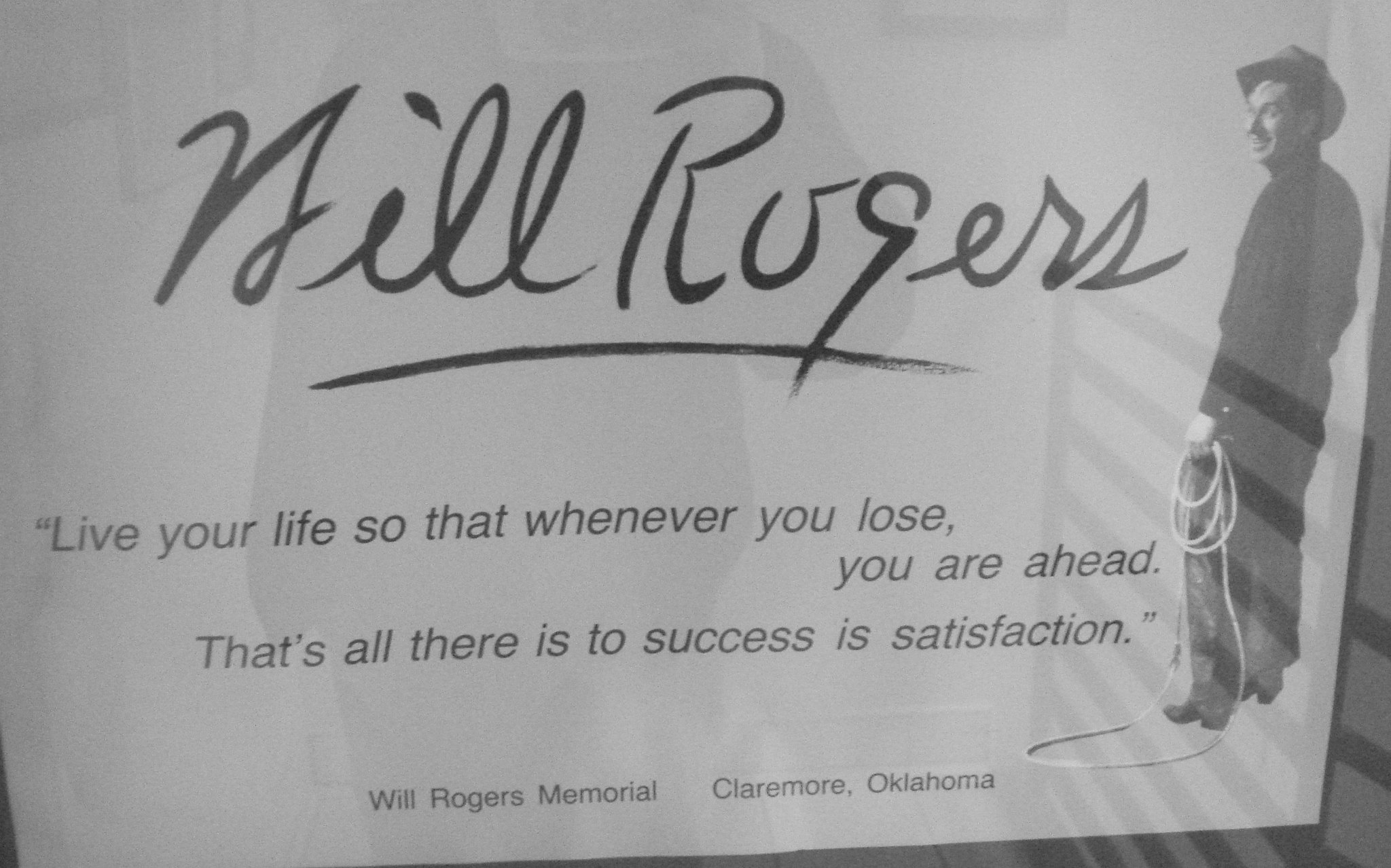This black-and-white photo captures a glossy, reflective poster centered in the frame. Prominently displayed at the top, "Will Rogers" is written in large, cursive print, underlined for emphasis. The central figure on the poster showcases a man, presumably a cowboy, characterized by his hat, black shirt, pants, and boots. He is positioned towards the left of the image but oriented somewhat towards the back, holding a coiled rope in his left hand.

The poster features a motivational quote from Will Rogers that reads, "Live your life so that whenever you lose, you are ahead. That's all there is to success is satisfaction." In smaller text below, it references the Will Rogers Memorial located in Claremore, Oklahoma. The background has a grayish hue with horizontal shadows that appear to be bars extending from the center towards the foreground. A faint reflection reveals the shadowy outline of the person taking the photograph, further contributing to the image's depth.